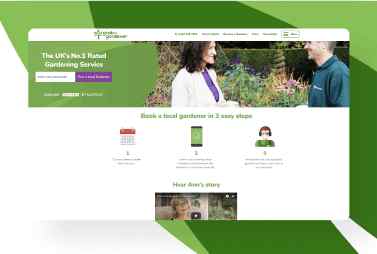This screenshot from a gardening service website features a blurry image with a predominantly green and white background. In the foreground, a woman in a white coat and blue t-shirt stands beside a man wearing a dark jersey. Both faces are not clearly visible. White text on the upper right or left side of the image reads, "The UK's number one gardening service." The bottom section of the image displays text that says, "In three easy steps," accompanied by three listed steps, though these are also blurred. The background of this section is white with green text, reinforcing the gardening theme of the website, albeit the details remain indistinct due to the blurriness.